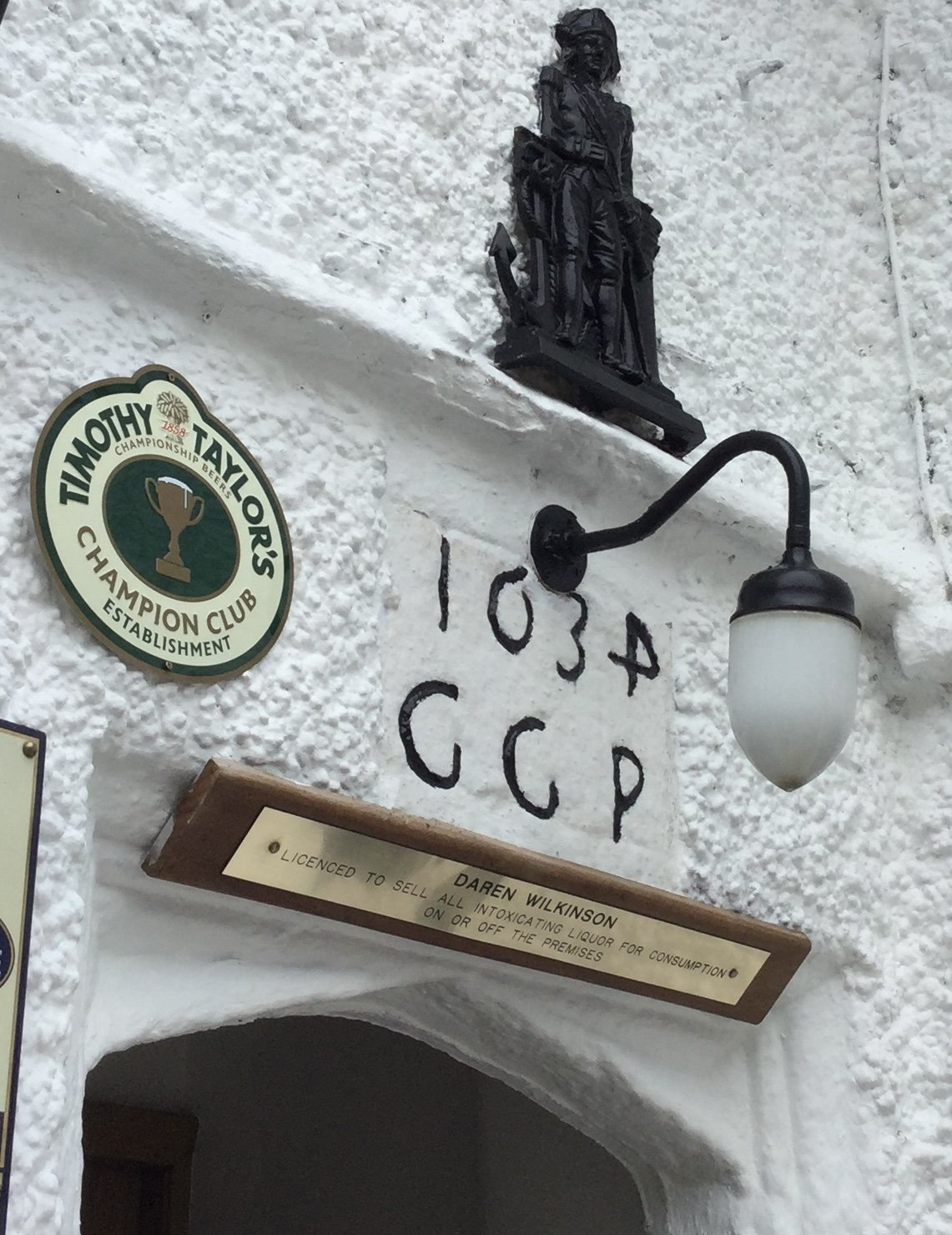The photograph captures the area above the front door of a white stucco building with a craggy texture. Centered at the top is a black 3D statue of a soldier seated on a chair, pinned to the wall. Below the statue, a black gooseneck lamp extends from the building, featuring a black iron bar and a white casing around the light. Directly beneath the lamp, black numbers and letters read "1034" with the "4" appearing backwards, and underneath, either "GGP" or "CCP." To the left of these letters and numbers, a round emblem with red, gold, yellow, and black colors proclaims "Timothy Taylor's Champion Club Establishment." Further down, there’s a wooden plaque with a gold bar inscribed in black, stating "Darren Wilkinson licensed to sell all intoxicating liquor for consumption on or off the premises." Just above the door frame, the details combine to create an intricate and richly described scene.